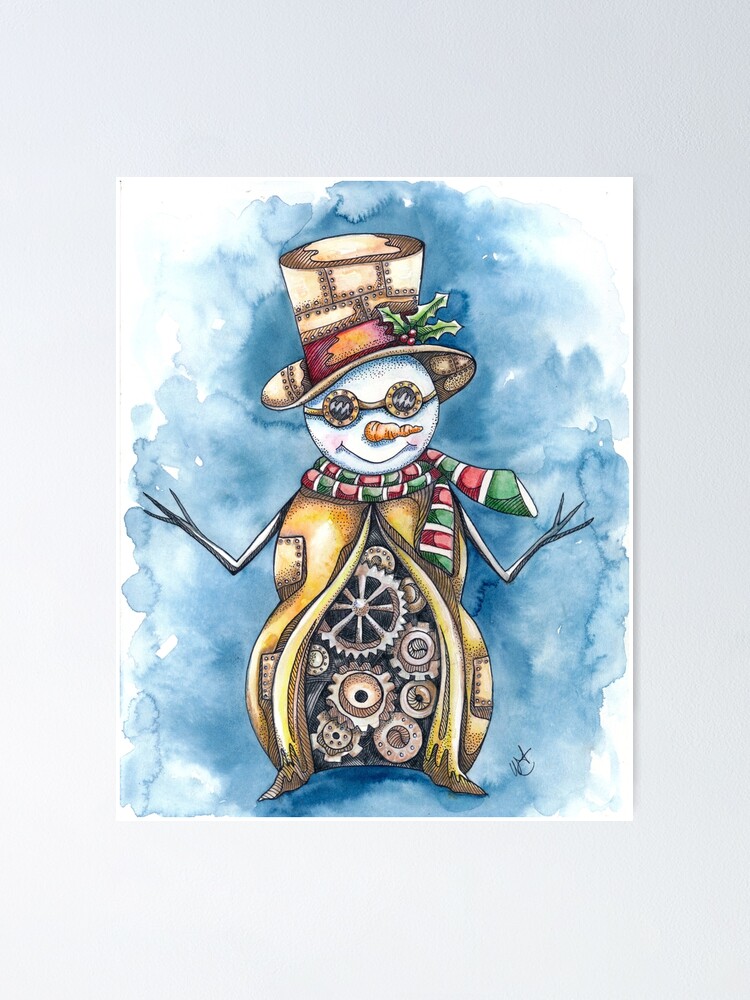This is a detailed watercolor painting of a steampunk-inspired snowman set against a backdrop that transitions from dark to light blue, seamlessly blending into a white border. The snowman stands out with its classic white snowball head, complete with a carrot nose and stick arms, both raised upwards. 

Adorning the snowman's head is a unique top hat, crafted to look like metal patches riveted together, with a red band at the bottom embellished with a sprig of holly and three red berries. Perched on the hat are welding goggles with detailed rivets. The snowman's black smile adds a whimsical touch to its mechanical appearance. 

Around its neck, a red, green, and white striped scarf is vividly wrapped, bringing a festive flair. The snowman's body is intriguingly designed to look as if it's made of metal, opening up in the middle to reveal a complex array of interconnected gears, with the largest gear prominent at the top and smaller gears arranged beneath it.

This artistic creation is set against a blue watercolor background that effortlessly fades into the natural white of the surrounding border, adding a dreamy, wintery ambiance to the steampunk snowman's striking and imaginative design.